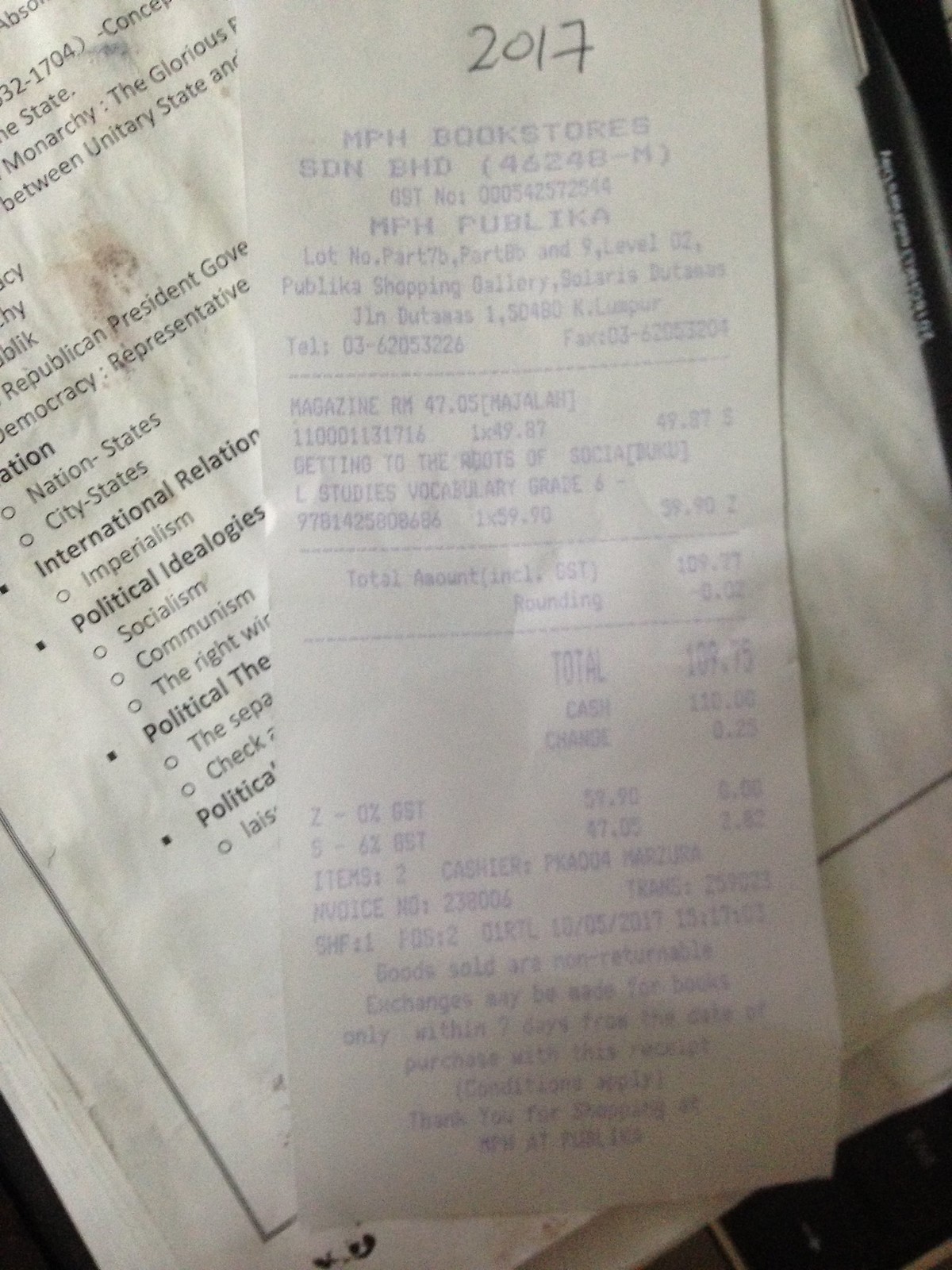The photograph is a detailed close-up of a receipt from MPH Bookstores, prominently displaying a handwritten note in black ink at the top indicating the year "2017." The receipt, printed in faint purple ink, stands out amid a backdrop of other documents, some of which feature noticeable water damage. Despite the faded and difficult-to-read text, it is discernible that this transaction took place in Kuala Lumpur, as indicated by the "K.LUMPUR" notation. Additionally, visible contact information includes a telephone and fax number. The total amount on the receipt is 109.75, which corresponds to the purchase of two items: one magazine (unspecified) and what appears to be an educational book titled "Getting to the Essentials of Social Studies Vocabulary, Grade 6," though parts of the title are blotted out. The receipt lies atop a wrinkled paper that lists geopolitical headers like "international relations" and "political ideologies," partially visible because it extends beyond the edges of the photograph.